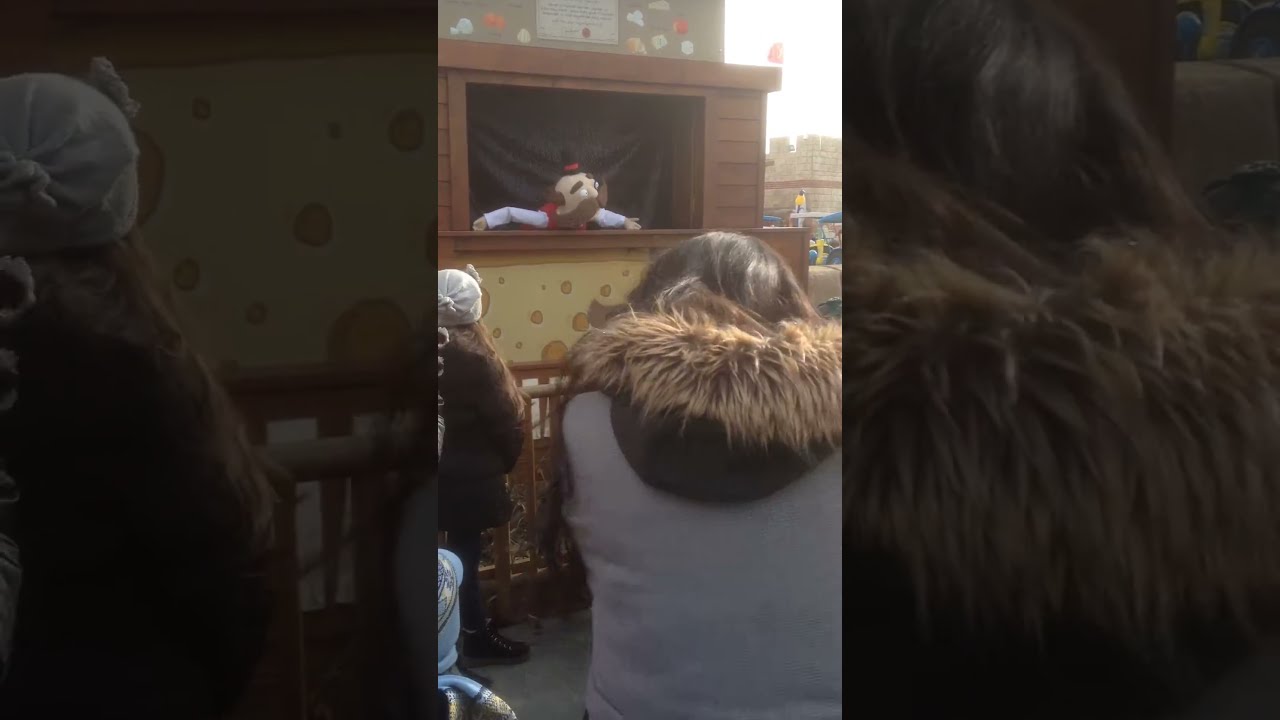This is a horizontally aligned rectangular image with thick black borders on the sides, revealing only a vertical strip in the center. The photograph captures an outdoor scene where three individuals are watching a marionette puppet show. The trio, all facing away from the camera, includes a child on the far left wearing a heavy red coat and having long brown hair, partially cut off by the black border. The middle figure appears to be a smaller child, dressed in dark clothing with a hood up. To the right stands a woman in a white coat with a fur-lined brown hood, and her long dark hair cascades down her left arm. They are gathered near a wooden structure that serves as the puppet stage. Above the stage, a painted character of a man with a black top hat, very long mustache, and mean eyebrows is visible. In the background, several flags flutter under a bright, glary white sky, hinting at a festive setting, possibly a carnival or festival. The overall image has a slightly overexposed, grayed-out appearance.